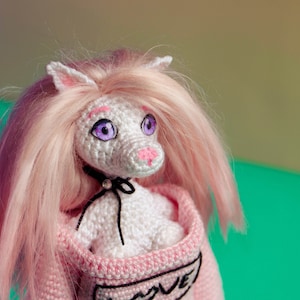The image features a small, intricately crocheted doll that closely resembles Miss Piggy from The Muppets. This homemade doll is crafted from very pale pink yarn and sports a charming black bow tied around its neck. The doll is seated in what appears to be a darker pink crocheted blanket or sweater. Prominently displayed on the front of this garment is a black-stitched rectangle with the word "LOVE" inscribed inside it. The doll is detailed with lavender eyes, a pink snout, and pink ears, which have a darker pink hue in their centers. Adding to its Miss Piggy likeness, the doll boasts a blonde wig with long hair cascading past its shoulders. The background is evenly split between a pastel green and a beige-cream color, providing a soft, complementary setting for the crocheted figure.